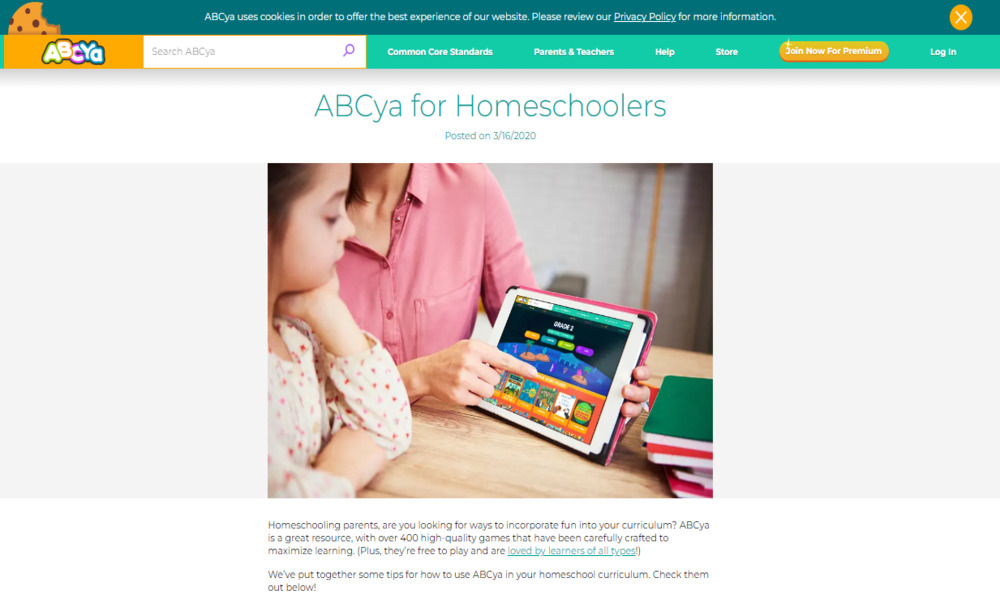Descriptive Caption: 

In the animated image, a half-eaten chocolate chip cookie is positioned in the very upper left corner. Below the cookie, an orange rectangle contains the block letters "ABCYA". Beside this rectangle is an image of a search bar with the text "search ABCYA" inside it. Below the search bar, the caption features the phrase "ABCya for Homeschoolers" in mixed uppercase and lowercase letters, along with the posting date "3-16-2020."

In the center of the image, a parent, wearing a pink shirt, holds an iPad, pointing to various educational content displayed on the screen, which includes different boxes, numbers, and letters. To the left, a child with dark hair, wearing a white and pink shirt, rests her chin in her hand, with her elbow on the table, attentively looking at the iPad.

The bottom part of the image emphasizes that the resource is intended "for Homeschoolers". In the upper right corner, there is an orange box with the clickable text "Join Now for Premium."